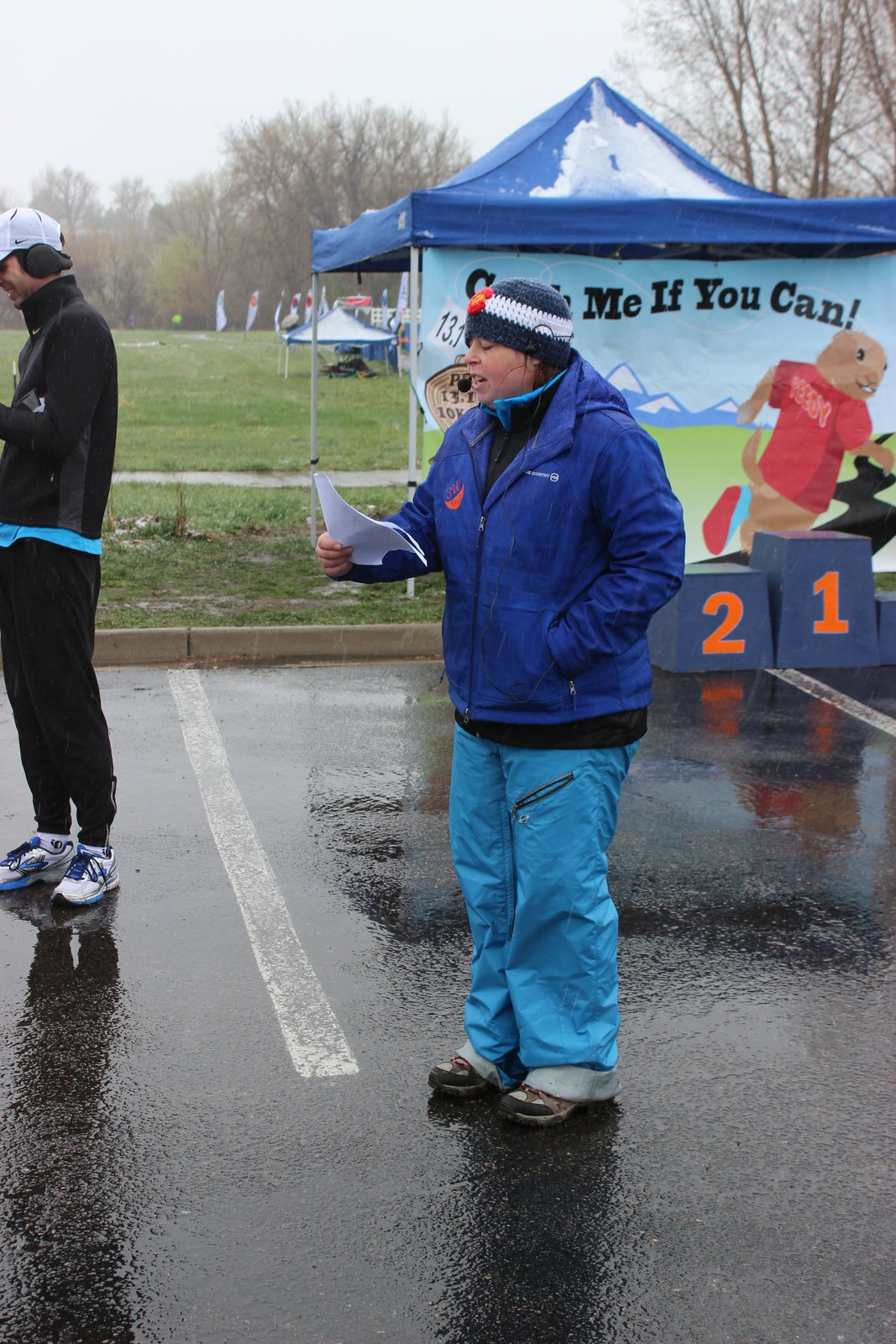The image captures a rainy, overcast day in an outdoor setting, specifically in a wet asphalt parking lot marked with white lines for parking spaces. In the foreground stands a woman, dressed in blue pants, a blue long-sleeved coat, a blue and white winter hat, holding some papers and looking down at them. To her left is a man, positioned between two parking spaces, wearing long black pants, black tennis shoes, a black long-sleeved shirt with a blue shirt peeking out underneath, a white ball cap, and black earmuffs. Both individuals appear to be engaged in conversation or reading from the papers. 

Behind them, on a grassy area, stands a blue pop-up tent canopy with a banner that reads "Catch me if you can," featuring an illustration of a sprinting red woodpecker or squirrel. Also visible are podiums for first, second, and cut-off view of the third place, emblazoned with numbers "2," "1," and "3" respectively. The backdrop includes flags and trees, providing a somewhat festive, race-like ambiance despite the absence of spectators due to the rain. The overall scene portrays a meticulous arrangement of colors ranging from various blues, blacks, whites, and greens, amidst the muted gray of the rainy day.